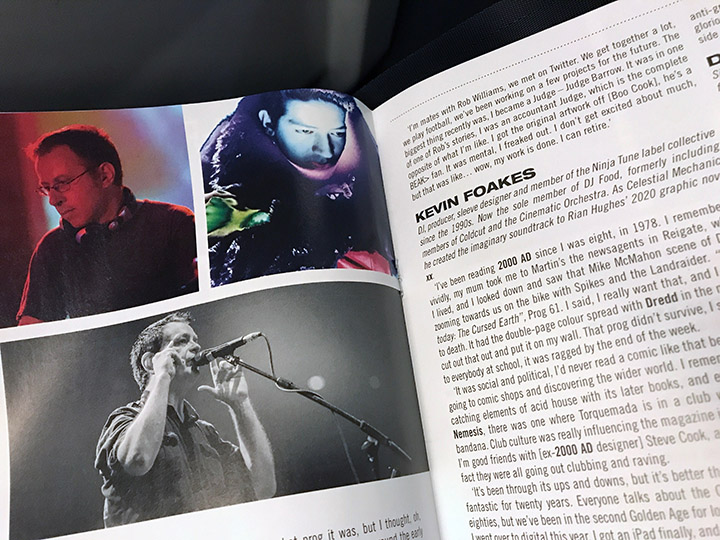The image depicts an open magazine spread. The left page features three photographs and some text: the top left photo shows a man with glasses looking to the left, providing a profile view of his face; the top right photo presents the same man with a glow beneath his face, creating a somewhat eerie effect; and the larger bottom photo captures him either talking or singing into a microphone. Below these pictures, partially cut-off black text is visible. The right page consists of an article about Kevin Folks. The article starts with a paragraph, followed by a heading that reads "Kevin Folks" in big black letters. It provides a mini-biography, describing him as a DJ, producer, and member of the Ninja Tune Label Collective since the 90s, as well as his association with DJ Food. There's additional detailed text about his career and accomplishments, but the page cuts off, suggesting the article continues further to the right. The magazine is tilted slightly, with the left page angled downward and the right page angled upward.